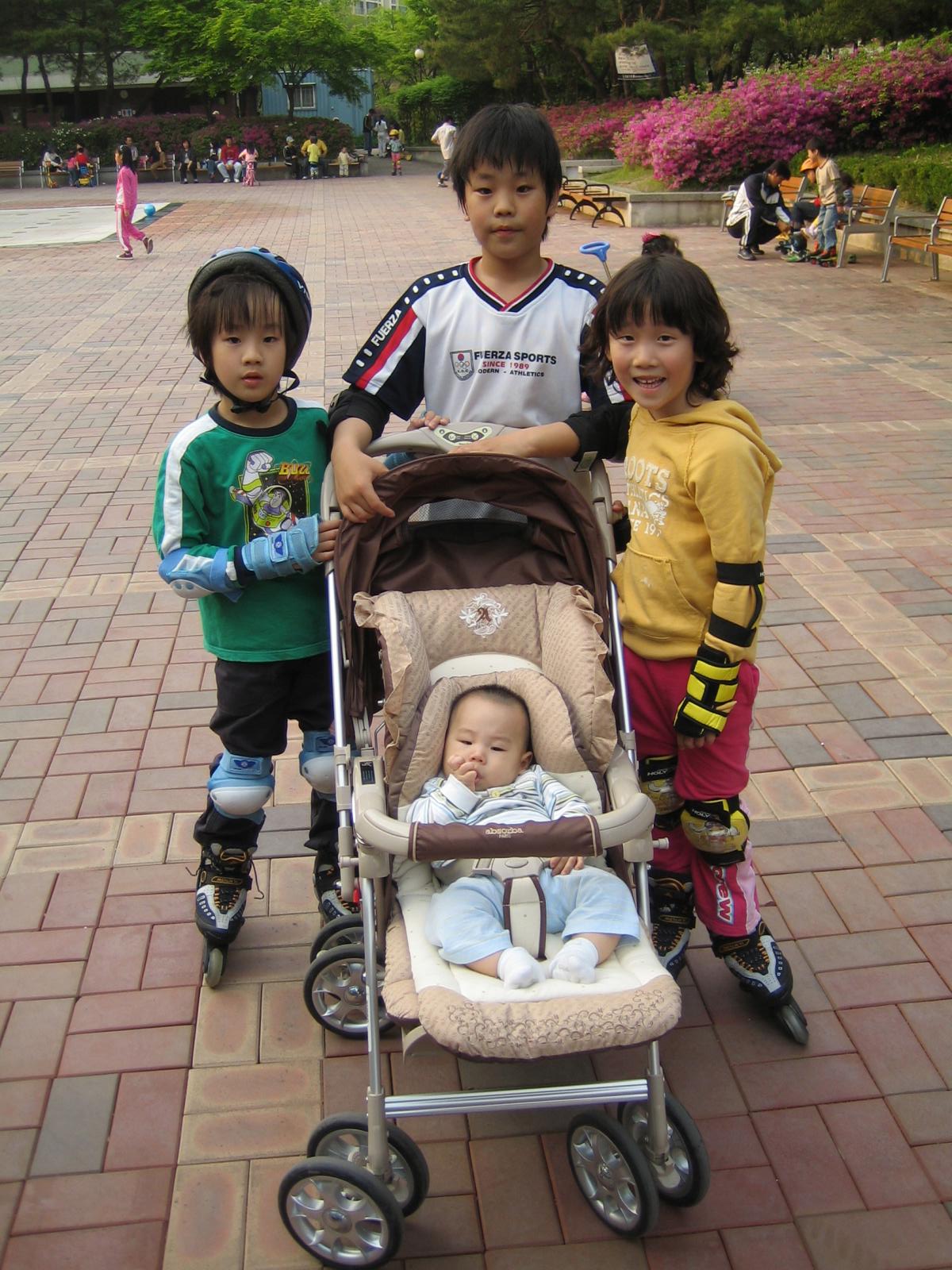In this detailed color photograph, captured in portrait orientation, we see a delightful family scene set in a public square with a red brick floor in various shades, some almost black. Central to the image are three Asian children standing in a semi-circle around a baby in a brown pushchair with tan cushions. The baby, dressed in blue, rests comfortably as the siblings engage with the stroller. The children on the right are a younger boy and girl, both equipped for rollerblading with knee pads, arm and wrist protection, and rollerblades. The girl sports a yellow long sleeve shirt, while the boy on the left, also in rollerblades, wears a green long sleeve shirt and a helmet. The slightly older boy in the middle, whose legs aren’t visible, wears a white jersey with blue sleeves and red and white stripes.

The scene is set against a stone retaining wall, not perfectly square, with 90-degree angles that encircles the area. In front of the wall are brown-planked, metal-framed benches occupied by people. Behind this wall, the landscape inclines slightly to the right, adorned with blooming pink and red bushes, likely azaleas, and green trees that add a vivid backdrop to this charming moment. The siblings hold onto different parts of the stroller, perhaps suggesting protective and playful interactions, making this a dynamically engaging family portrait in a tranquil park setting.